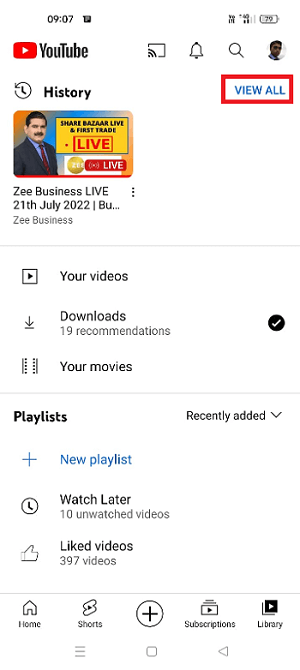Screenshot of YouTube App Interface

The screenshot showcases the main interface of the YouTube app on a smartphone. The timestamp in the top right corner indicates 09:07, and the battery is approximately at 70%. 

At the uppermost section, the YouTube logo is prominently displayed. To the right of the logo are several icons: a bell symbolizing notifications, a magnifying glass for search functionality, and a user profile picture.

Positioned below this row is a horizontal menu with a "View All" tab flanked by a "History" tab on the left. Beneath this menu is a video thumbnail titled "Share Bizarre Live and First Trade Live. Live", from Z Business, dated 21st July 2022. This entry is followed by an options menu represented by three vertical dots.

Further down, there are sections labeled "Your Videos", "Downloads", and "Your Movies". Within the "Downloads" section, there is a checkmark indicating 19 recommendations. 

The "Playlists" section is also visible, featuring a drop-down arrow labeled "Recently Added". Below it, users can create a new playlist with a plus icon, or manage their "Watch Later" list which has a clock icon. Additionally, "Liked Videos" are displayed with a thumbs-up icon and currently indicate a total of 397 likes.

At the very bottom of the interface, navigation tabs are present: "Home", "Shorts", a plus symbol, "Subscriptions", and "Library". Just below these tabs, there is a hamburger menu icon, a home button, and an arrow pointing left for back navigation.

This detailed depiction captures the various functionalities and sections available on the YouTube app, providing a comprehensive view of a user’s home screen.